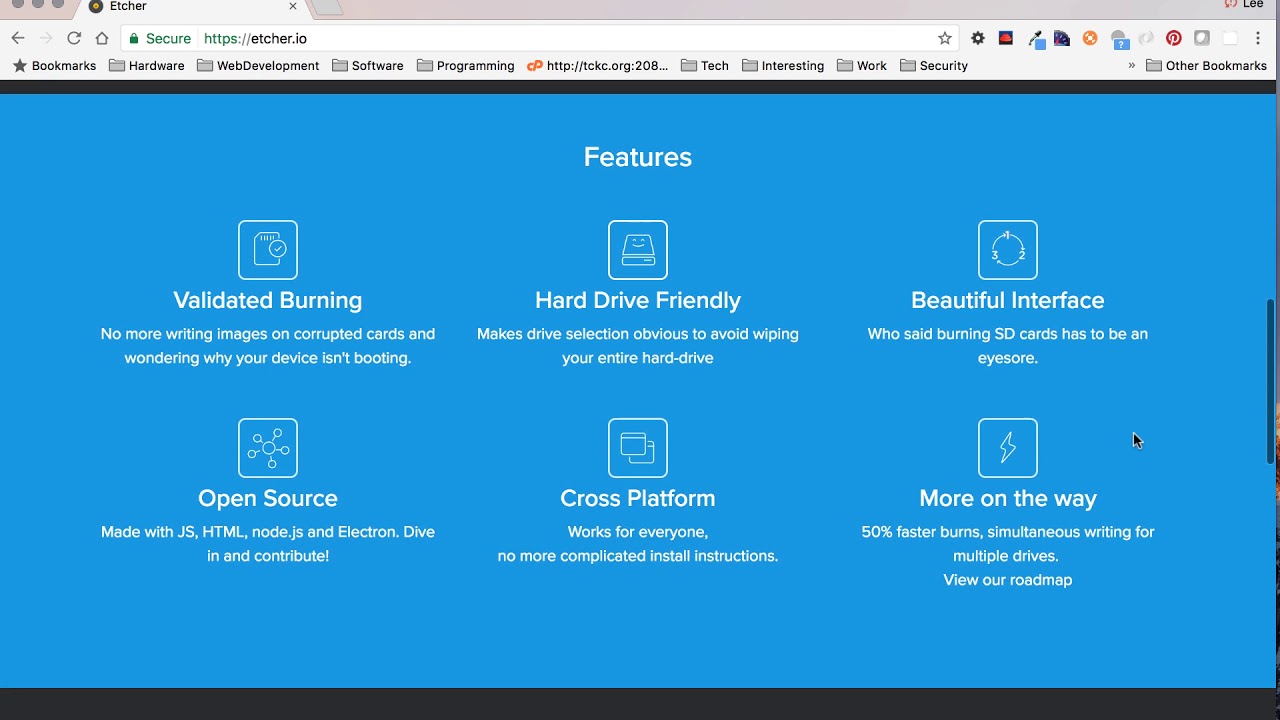A screenshot taken on a Mac web browser with a partially visible top toolbar, showing three darker icons against a white or gray background. The active tab is labeled "Etcher" in black text, with an adjacent gray bar extending to the right, where the user name "Lee" is faintly visible on the upper right-hand side. Below the toolbar, the light gray bookmarks bar is displayed. The primary content of the screenshot features a baby blue background with white text that reads "Features" at the top center. Below this title, the screen displays a three-by-two grid layout with the following headers: "Validating Burning," "Hard drive friendly," "A beautiful interface," "Open source," "HTML," and "Cross platform." Underneath each header, smaller white text is present but unreadable in this image. The phrase "more on the way" appears next to "Cross platform," with a mouse cursor positioned to the right of this text. Additionally, a darker vertical element resembling a scroll bar is visible on the right-hand side of the screen.